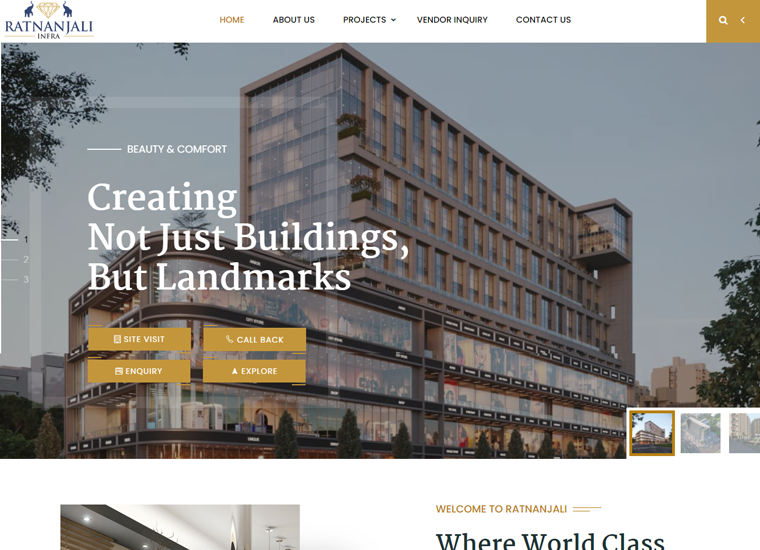The image is a partially framed photograph with a bottom and top border of white, each about two inches and one inch respectively. The central portion of the image is occupied by an elaborate picture.

In the top left corner, there is an outline of a gold diamond shape. Flanking the diamond on both sides are silhouettes of elephants with their trunks raised. Underneath this in bold, all-capital, blue lettering reads "RATNANJALI." Below this title, in smaller blue capital letters, it says "INFRA." Extending horizontally from these words are two gold lines about one inch long each. 

Approximately two inches to the right, in gold, is the word "Home." Following this, in blue, are the words: "About Us," "Projects," "Vendor Inquiry," and "Contact Us." Toward the right side of the picture, there is a gold square containing a white search icon on the left side, accompanied by a greater-than sign pointing left.

The bottom section of the picture shows a clear blue sky and a green tree in the top left corner as well as another green tree in the bottom right corner. Dominating this section is a large two-story building with extensive windows. Extending upward from the top of the building, about two inches from the left, is an additional four-story structure with more windows.

On the left side of this structure, approximately two inches from the top and one inch from the left, are the words "Beauty and Comfort" in small white letters. Following this, in bold white text, it says "Creating," followed by the phrases "not just Buildings," "but Landmarks" in smaller white text. 

Below this motivational quote, there are four gold tabs arranged in a two-by-two grid, each with white lettering. In the bottom right corner, there are three small clickable images, with the first (on the left) highlighted with a gold trim, while the other two appear gray and faded.

Just below these, in the white bottom margin, you can see the top of another image, showing part of a white and gray ceiling. In the central white area, the text, "Welcome to Ratna Jolly" appears in gold, followed by the bold black text "World Class," but the image cuts off before the reader can see the rest.

This caption ensures all elements of the image are described with attention to precise details and positioning.